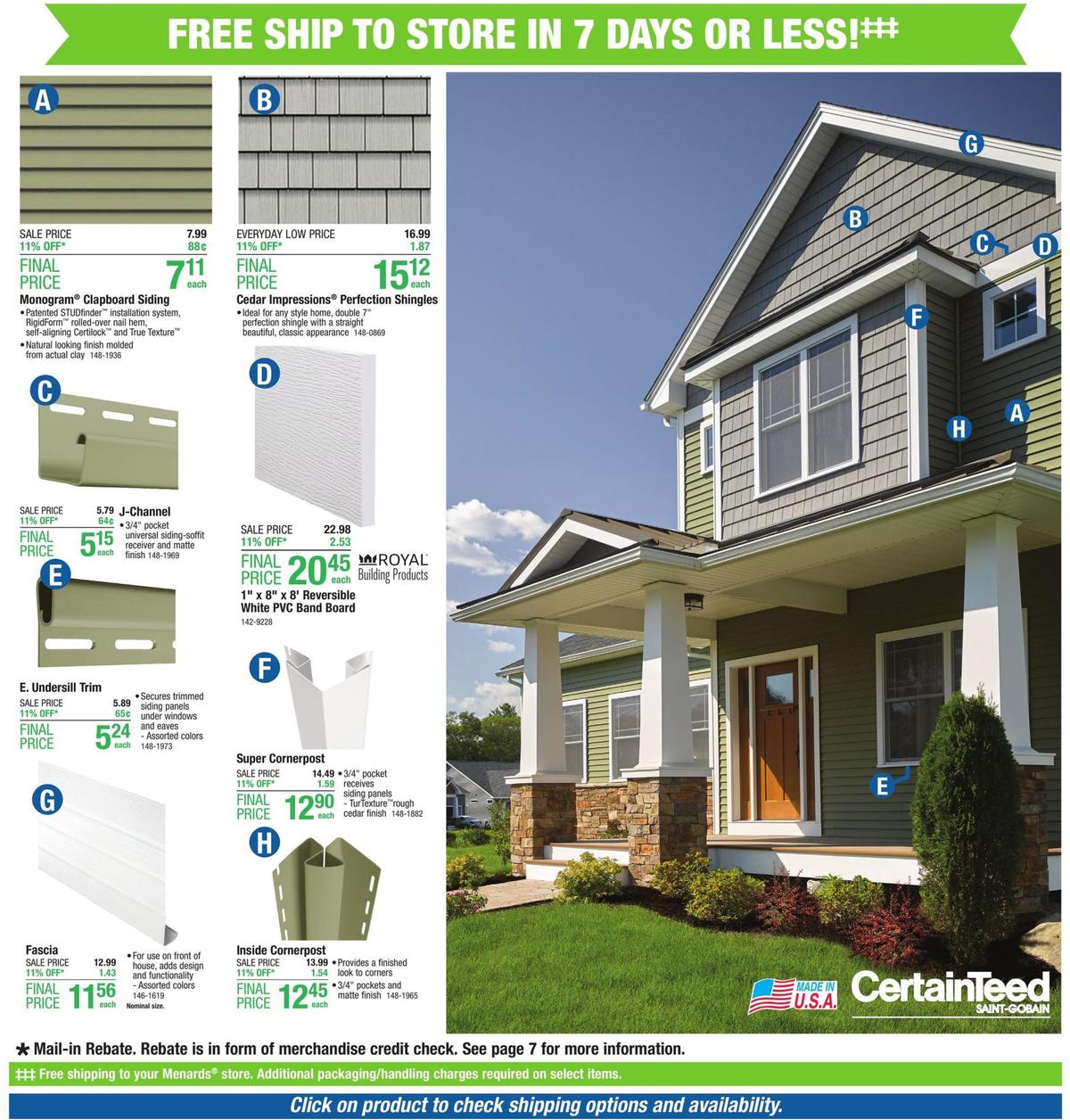**Advertisement for CertainTeed Roofing and Siding**

At the top of the advertisement, a green banner with bold white text promotes "Free Ship to Store in 7 Days or Less." The ad is for CertainTeed, a company specializing in roofing and siding services.

The right section features a detailed picture of a modern two-story suburban house, showcasing various siding and roofing options. Icons and letters are mapped onto different parts of the house, correlating with specific products the company offers.

On the left side of the ad, these letters are matched with corresponding siding options and images. For instance:
- **Letter A**: Monogram Clapboard Siding
- **Letter B**: Cedar Impressions Perfection Shingles, illustrated as gray shingles at the top of the house.

Additional options are depicted, such as:
- J-Channel Receivers for gutters
- Reversible White PVC Band Board
- Under-sill Trim
- Corner Posts for exterior jutting corners
- Inside Corner Posts for a finished look on interior corners

At the bottom of the page, various customer benefits are highlighted:
- A mail-in rebate available as a merchandise credit check
- Free shipping to your Menard store, with a note that additional packaging and handling charges may apply to selected items.

The ad concludes with a blue background banner with white text, stating, "Click on product to check shipping options and availability."